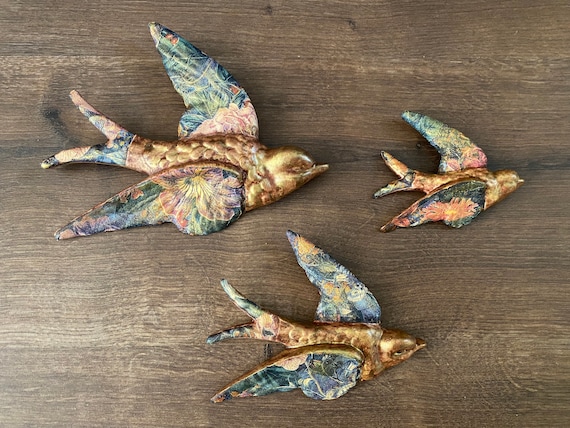This is an overhead view of three retro-style bird figurines on a dark wooden table. The figurines, varying in size from large to medium and small, are made of a metal with a goldish-bronze body. Each bird features intricate floral patterns painted on their wings and tail feathers, showcasing a vibrant spectrum of colors including greens, reds, blues, pinks, yellows, and purples. The largest bird, positioned at the top left, has a forked tail and its wings and tail display an array of floral designs. Directly in front of the large bird is the smallest bird, which mirrors the same gold body and colorful wing patterns, with a forked tail similar to the large bird. Between the two, situated at the bottom of the image, is the medium-sized bird. Like the others, it has a gold body with floral patterns painted on its wings and tail feathers. All three figurines share the same basic design elements with their outstretched wings and detailed, colorful ornamentation, creating a cohesive and decorative trio.